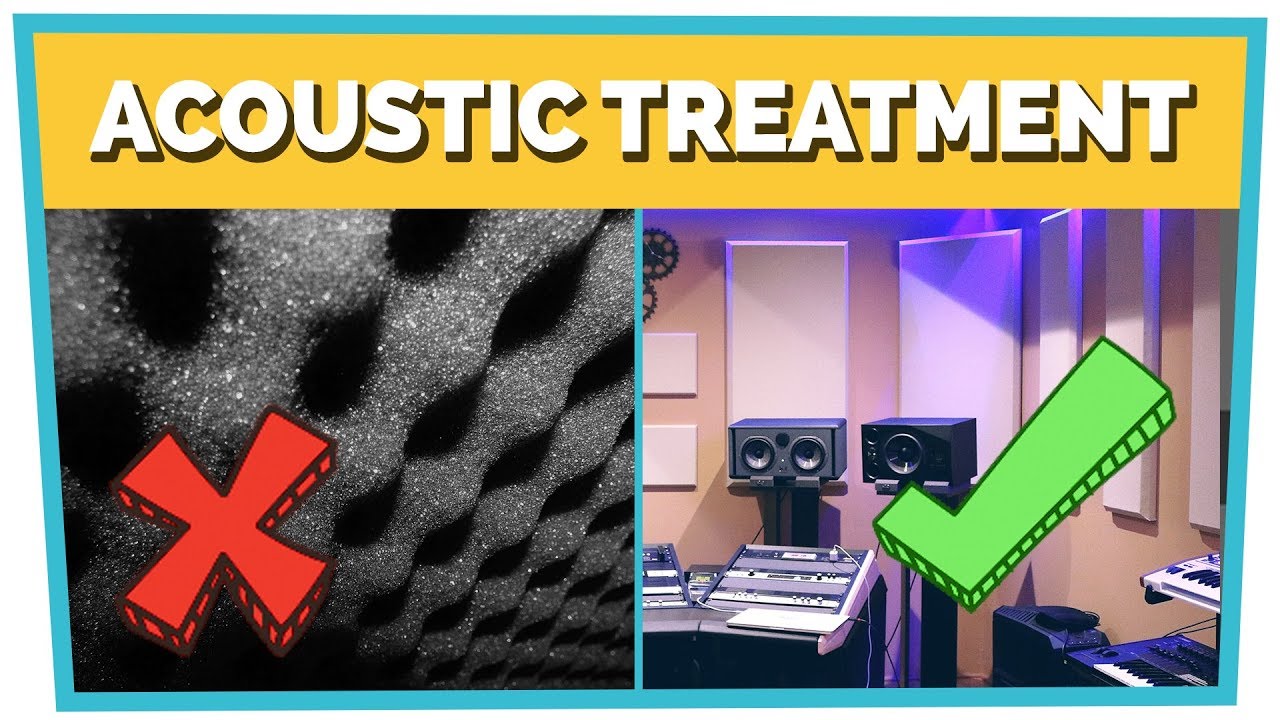The image is a skewed rectangular graphic with a light blue border. At the top, a yellow bar with white capital letters, featuring a solid black drop shadow, reads "Acoustic Treatment." In the left photo, black foam commonly used for soundproofing walls in studios is depicted with a red X at the bottom left corner, indicating it's not the recommended solution for acoustic treatment. The right photo showcases a music studio filled with speakers, a table with music equipment, a piano, and white acoustic panels mounted on the walls. A green check mark is placed on the bottom right corner of this photo, signifying this setup as the correct method for acoustic treatment.